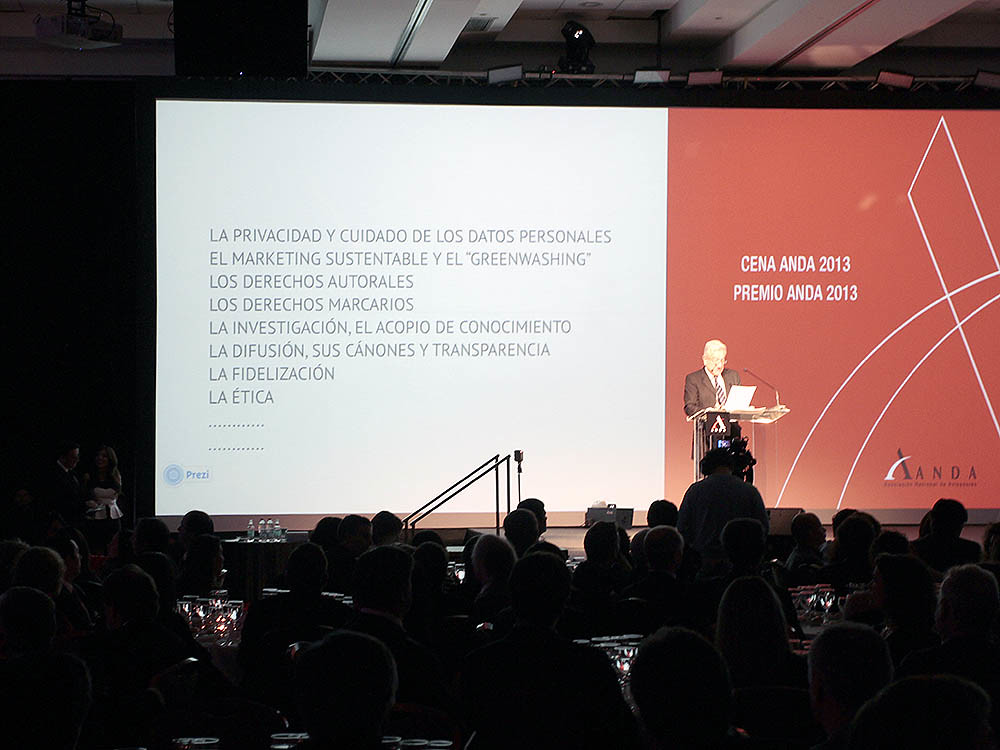An older man, distinguished by his gray hair and glasses, stands on a stage in a conference hall, giving a lecture from a transparent plexiglass podium equipped with a microphone. Wearing a suit and tie, he holds a piece of paper and reads as he addresses the audience, their heads dimly lit in the background. Behind him, a projection displays text in Spanish or possibly Portuguese. The screen features an orange background on the right and light gray text on the left, with prominent words including "Premio ANDA 2013" and a logo resembling an "X." The year 2013 is highlighted, and the event appears to be sponsored by ANDA. The audience, likely students or professionals, includes individuals using laptops or tablets, though the details are obscured by the dim lighting.